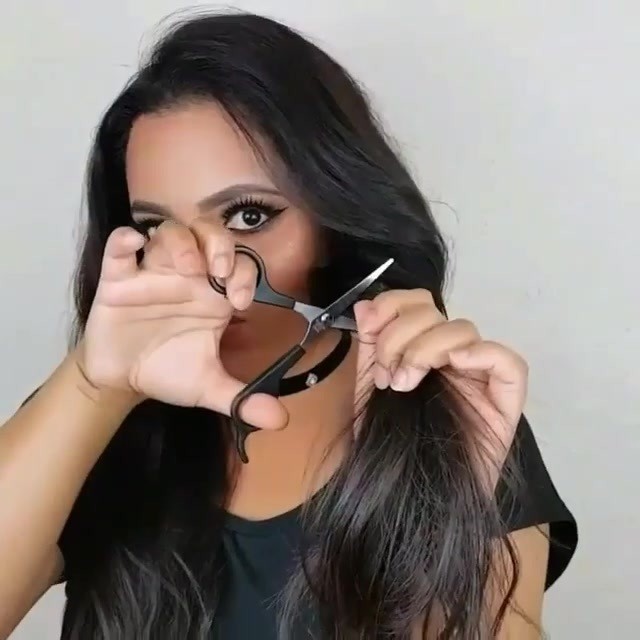This photograph features a young woman with long, dark brown hair, seemingly of Hispanic or Latina descent, in the act of appearing to cut her own hair. She faces the camera with her head slightly tilted to the right, her expression serious, and her right hand holding a pair of short-bladed scissors with dark brown plastic handles. The scissors, intriguingly held backwards with a loop extending off her thumb, block much of her face, partially obscuring her mouth which is set in a neutral line. Her left hand grips a section of her hair, extending it out in front of her with sharply bent elbows. She is adorned in heavy makeup, featuring long eyelashes, black mascara, and bold eyeliner that wings out in a cat-eye pattern. Her thick, dark eyebrows frame her expressive eyes. She is dressed in a short-sleeved black t-shirt and wears a choker necklace with a small diamond pendant around her neck. The background of the image is plain white, emphasizing the detailed elements and posing of the subject. The overall composition and the somewhat blurred facial features suggest that the photograph might be an AI-generated image, adding a layer of intrigue to the scenario depicted.